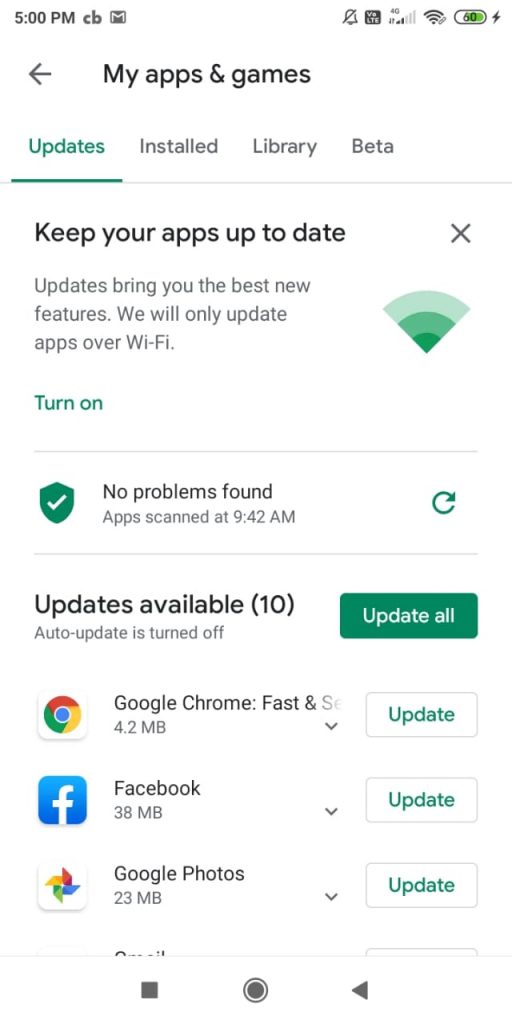The image features a user interface with a clean white background. At the top, there is a timestamp reading "5:00 p.m." On the top-left corner, a label "CB" is visible next to a small square containing the letter "M." Just below that, a left arrow icon is accompanied by the text "My apps & games."

This section is divided into tabs with the labels "Updates," "Installed," "Library," and "Beta," with the "Updates" tab highlighted in green and underlined. Beneath this, there is a message reading "Keep your apps up to date" with an "X" icon on the right side to dismiss the notification. The accompanying text explains, "Updates bring you the best new features. We will only update apps over Wi-Fi." Following this, a prominent green button labeled "Turn on" is displayed next to a small, green triangle with various green stripes.

A horizontal line separates this section from the next, featuring a green shield icon with a white checkmark and the text "No problems found. Apps scanned at 9:42 a.m." A return arrow and another horizontal line follow.

Further down, the section "Updates available" indicates that 10 apps need updates, and a note mentions that "Auto-update is turned off." Beneath this, a large green button marked "Update all" is presented.

Below this button, the names of individual apps appear, each with downward arrows and "Update" buttons next to them:
- "Google Chrome: Fast & Secure" 
- "Facebook"
- "Google Photos"

The bottom of the interface features a navigation bar with three icons – a square, a circle, and a triangle, all set against a white background.